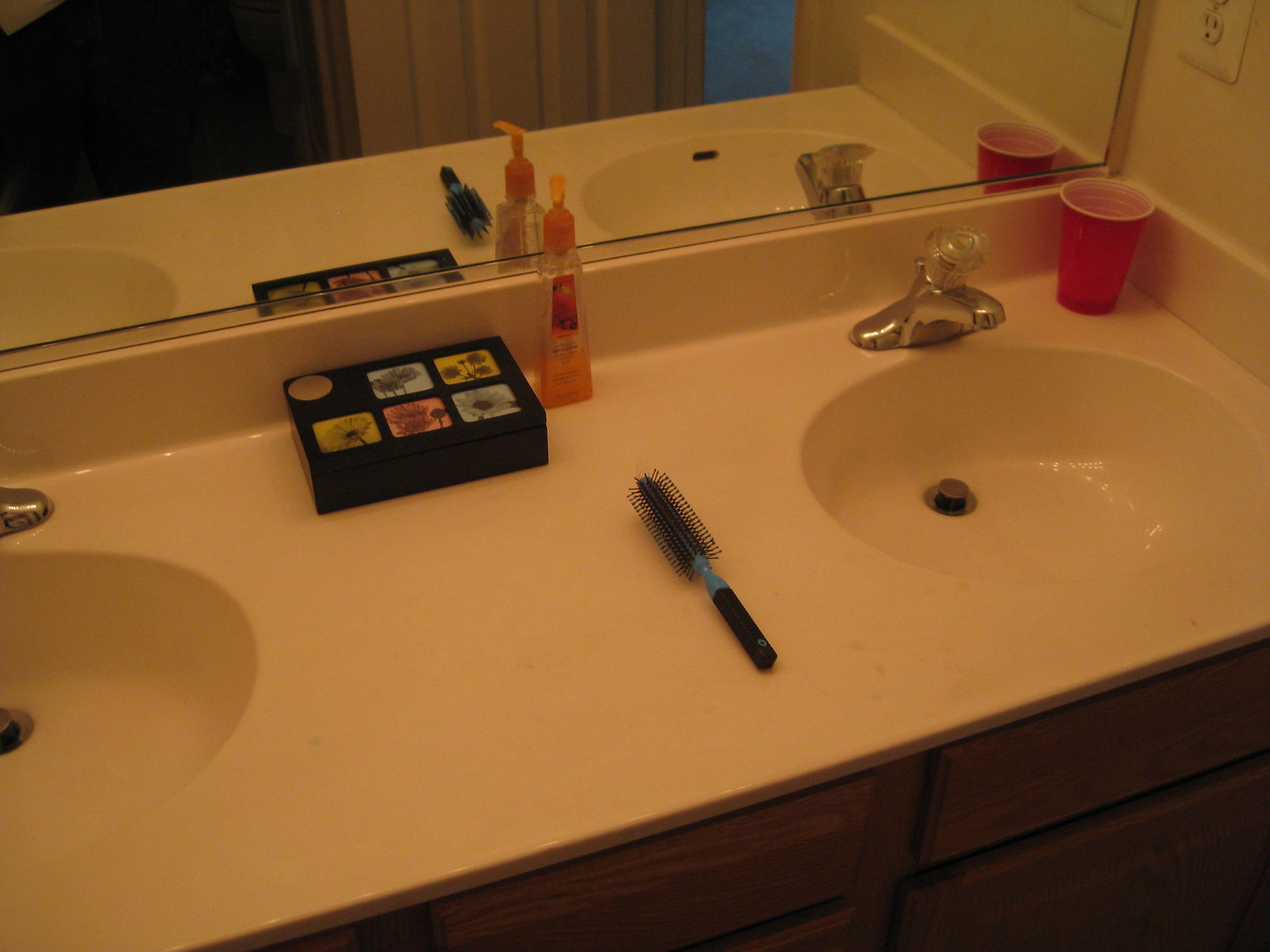This photograph captures a double-sink setup in a bathroom, taken in landscape orientation. The sink unit features two white, built-in basins set into a white countertop. The front face of the countertop is adorned with a wooden façade, lined with multiple drawers. 

In the background, a large mirror spans the width of the sinks, reflecting an open door behind the photographer. In the top right corner, a white electrical outlet is visible, appearing to have a single socket shown but likely housing another above it. Directly below this outlet, a red Solo cup is positioned against the corner of the sink, as seen in the mirror's reflection.

The right-hand sink is equipped with a stainless steel faucet that has a clear, knob-style handle. The drain is in an opened position. Between the two sinks, there is a rounded brush with a black handle and blue base, characterized by tiny, hair-like bristles. Behind this brush, almost touching the mirror, is a soap bottle containing a liquid that appears to be either orange or pink. Adjacent to the soap bottle is a rectangular black box with six visible compartments or images on its front. The left sink is partially cropped out of the frame, concluding the detailed contents of the photograph.